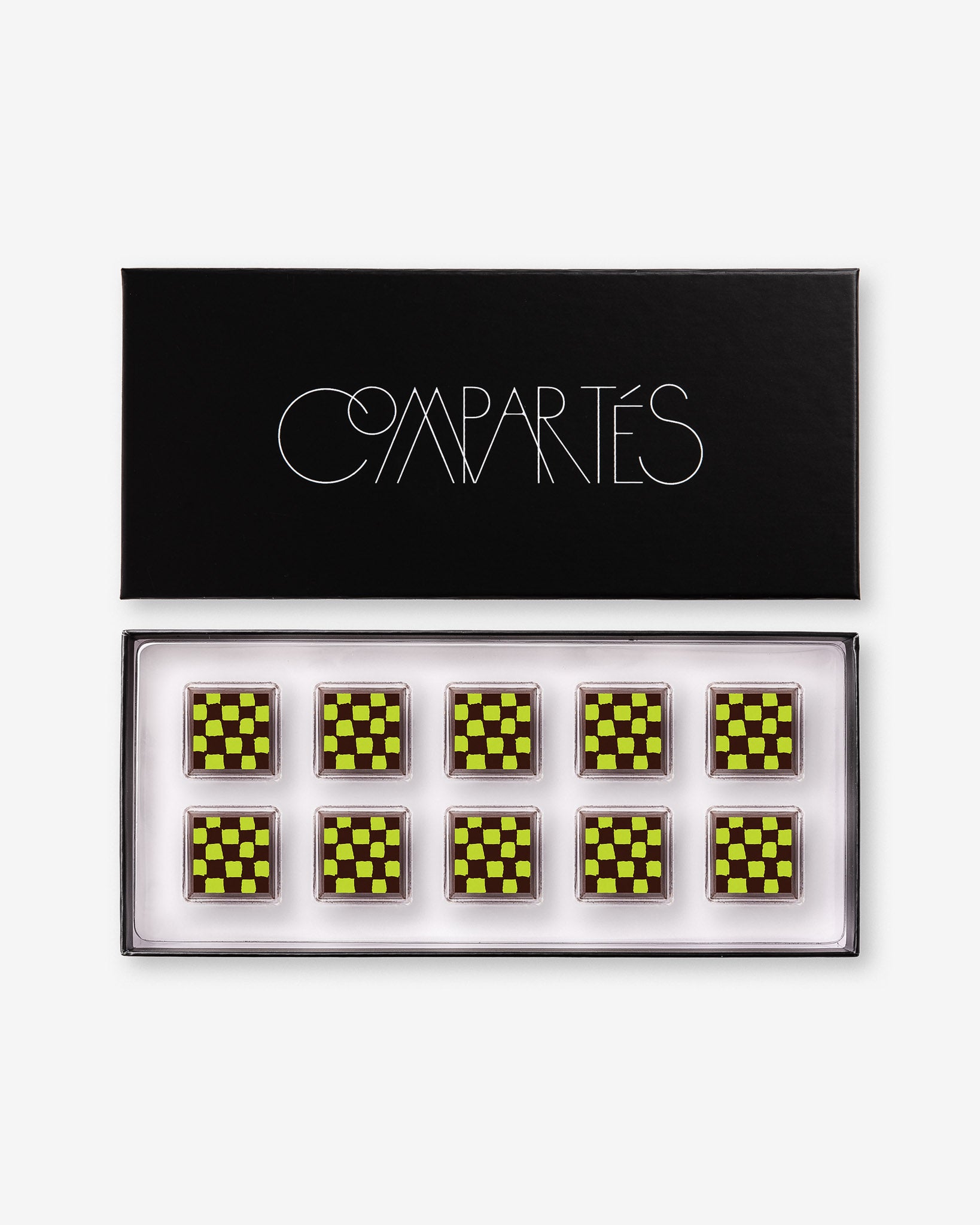The image showcases a luxurious arrangement of Compartés chocolates, elegantly displayed in a sophisticated container. The container holds ten exquisite chocolates, organized in two rows of five, each meticulously crafted with a distinctive black and lime green checkerboard pattern. These chocolates are set into precise indentations within the case, accentuating their high quality and artisanal nature. The case itself is adorned with an eye-catching lid featuring the brand name "Compartés" in a stylish, custom white font on a black background. This unique font evokes a vintage 1920s aesthetic, with elements like the "M" resembling three peaks and other letters contributing to its quirky charm. The setting is further framed by a light off-white backdrop with faint lines, possibly indicating a digital overlay, while the outer edge of the image is encircled by a subtle light gray background.